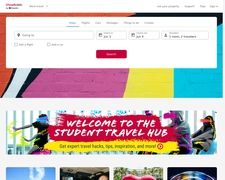Screenshot of a Student Travel Website: The image depicts the entire webpage of a student travel-focused site, albeit with the text being heavily pixelated and difficult to discern due to extreme zoom-out. At the top of the page, there appears to be a form intended for inputting travel details, resembling what you might find on an airline's booking platform. Users likely enter departure and destination locations along with travel dates and other pertinent information for search purposes.

Midway through the page, a prominent banner reads "Welcome to the Student Travel Hub," reinforcing the travel-centered theme of the site. The background is visually engaging, featuring people in vibrant hues dancing, with colorful overlays obscuring their eyes. This adds a lively and energetic aesthetic to the page. Dominant colors in the background include shades of reddish-orange, white, black, hot pink, yellow, and bright blue, creating a dynamic and visually appealing layout that draws the eye to various elements of the site.